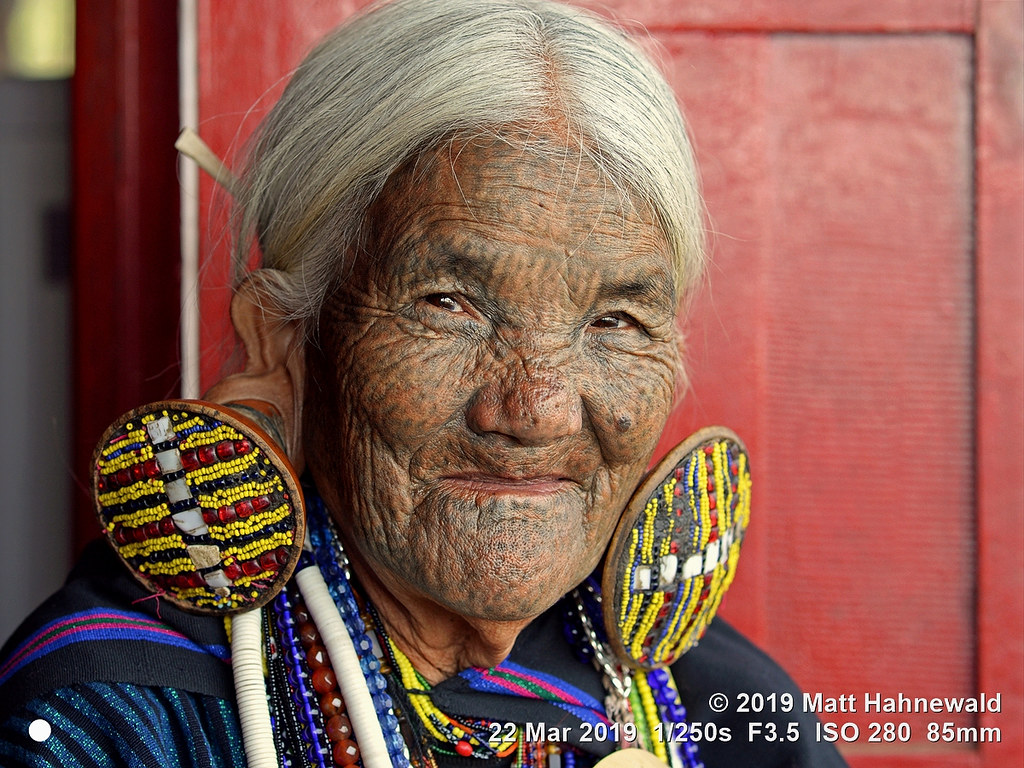This photograph captures an elderly woman with a deeply wrinkled face and dark skin, adorned with intricate tattoos consisting of black dots covering her face. She has long, white hair parted down the middle, cascading towards the back. Her dark brown eyes hold a depth of experience, and she is ornamented with prominent gauge earrings that have stretched her earlobes. These elaborate earrings feature intricate adornments with yellow beads, white, and red gems. She is dressed in an attire rich with cultural significance, including various necklaces made of blue, red, and white beads. Over her right shoulder, a strap extends across her body, hinting at traditional garments. She wears something blue and there are embroidered fabric pieces on either side of her head, with brown outlines and vibrant colored lines of red, yellow, and blue. Behind her, you can see a red shutter or door, adding a splash of color to the setting. This woman's appearance, jewelry, and attire suggest she is a respected member of a tribal community, possibly from Central or South America. The photograph is signed "2019 Matt Honwald" with additional details marking the date "22 March, 2019," and the camera settings "1/250s F3.5 ISO 280 85 mm" in the bottom right corner.